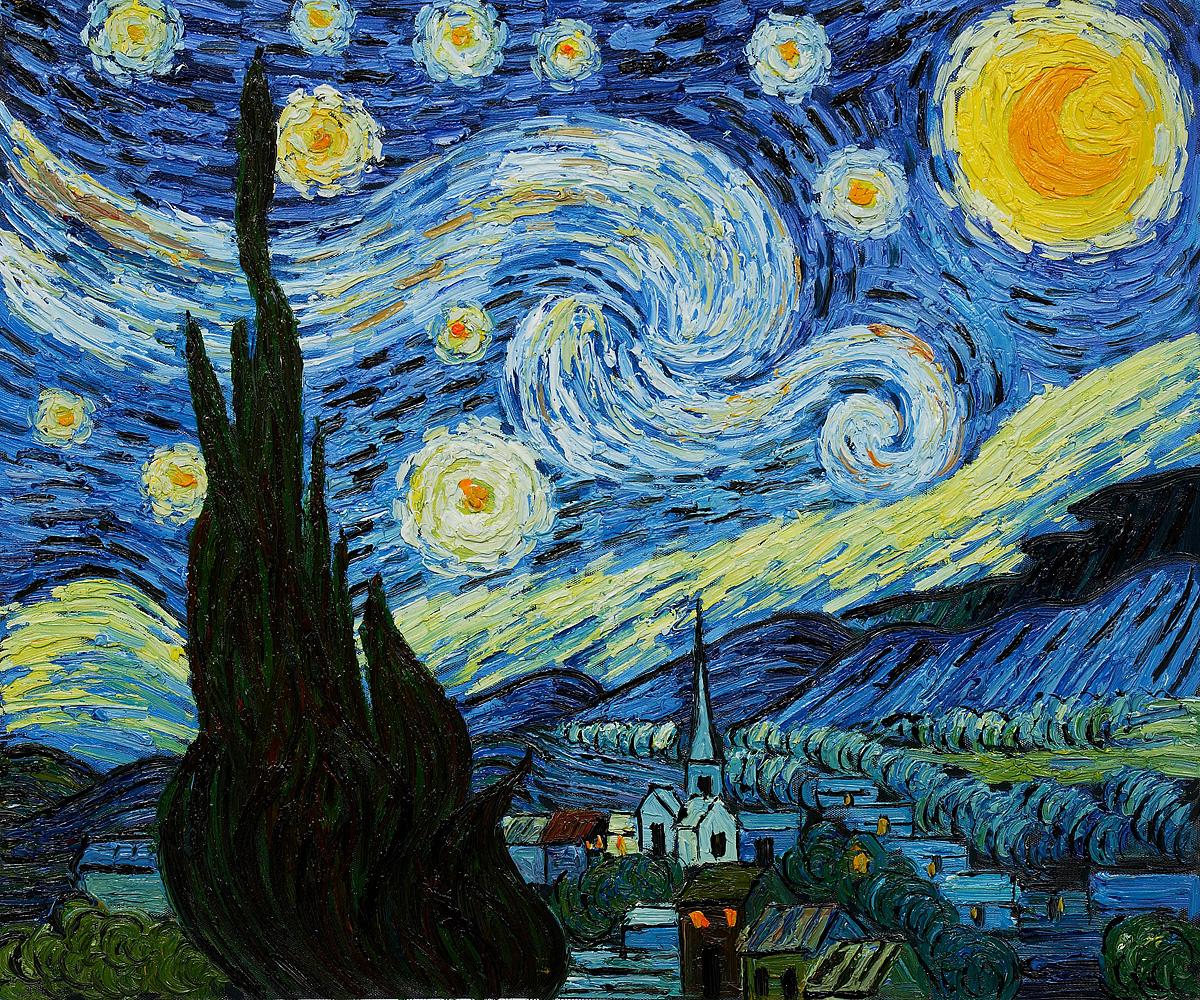The image depicts Vincent van Gogh's iconic painting "Starry Night." This Impressionist masterpiece showcases a vibrant array of colors dominated by shades of blue, highlighted with yellow, orange, white, and interspersed with dark areas of black, dark green, and deep blues. The upper portion of the painting, about one-half to one-third, features a dynamic evening sky filled with swirling patterns of blue representing clouds and winds. This starry sky is dotted with bright yellow stars encircled by white, and the upper right-hand corner features a radiant full moon, edged in white with a dark orange crescent at its center. Below the mesmerizing sky, rolling hills or mountains form the middle section, leading down to a quaint town nestled in the lower third of the painting. This town includes various buildings, trees, and a prominent church steeple slightly off-center to the right. Dominating the left foreground is a towering, dark cypress tree, anchoring the composition with its vertical formality against the whimsical, flowing movement of the sky. The overall effect is a vivid, swirling depiction of a night sky over a peaceful village, enveloped in a sense of motion and color that captures Van Gogh's masterful interpretation of the Impressionist style.